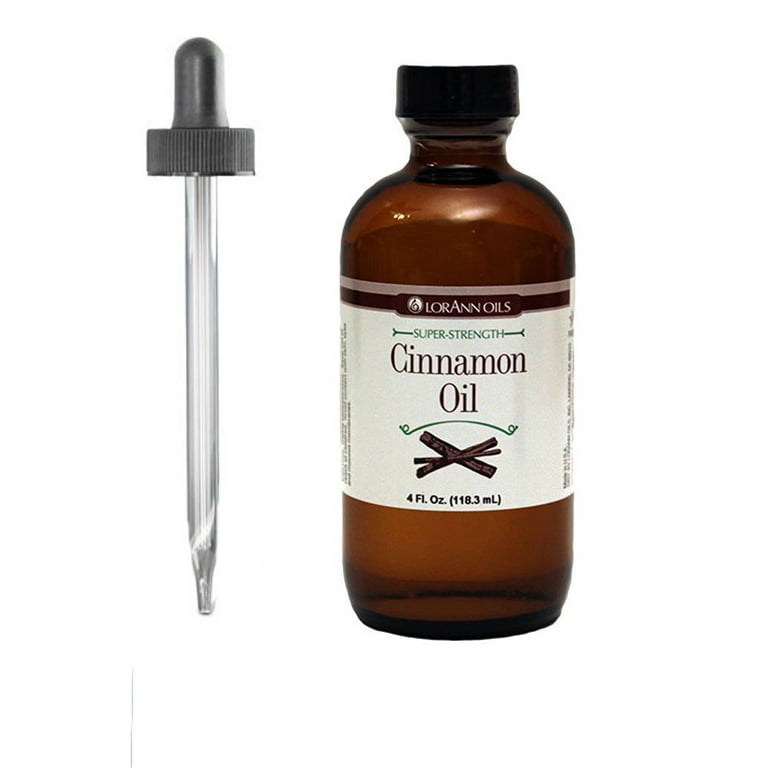This product photo showcases a bottle of LorAnn Oils' Super Strength Cinnamon Oil. The main focus is on a small, brown-toned amber bottle with a black top and a dropper situated to its left. The dropper, depicted upright as if held, features a black squeezy top and a clear tube. The bottle's simple, off-white label prominently displays the product name, "Super Strength Cinnamon Oil," in green with a decorative swoop below the title. Beneath this swoop, an illustration of three cinnamon sticks is clearly visible. At the bottom of the label, the volume is indicated: "4 fluid ounces (118.3 milliliters)." The right and left edges of the label, while not fully readable, contain additional information. The entire image appears to have been edited to remove the surface, leaving just the products in focus.